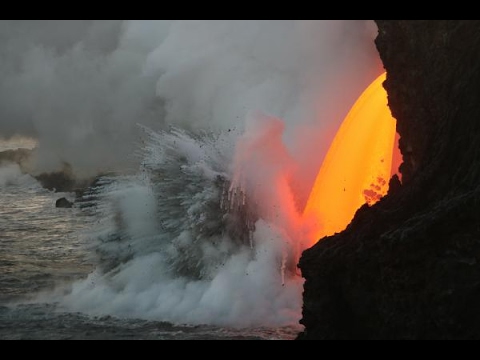This striking photograph captures a dramatic interaction between molten lava and ocean water in the Hawaiian Islands. A vivid, red-hot stream of lava cascades from the rough, black volcanic cliffside into the sea, creating a breathtaking scene. Upon contact with the cool ocean water, the intense heat causes a violent reaction, producing thick, white steam and bursts of debris that shoot outwards. The steam and vapor rise up like voluminous, cottony clouds, dominating the center and upper left part of the image. To the right, the rugged black cliffside stands in stark contrast to the chaotic, boiling water below. The raw power and natural beauty of this moment are encapsulated in the massive cloud of steam and scattered fragments, making it a memorable and awe-inspiring sight.